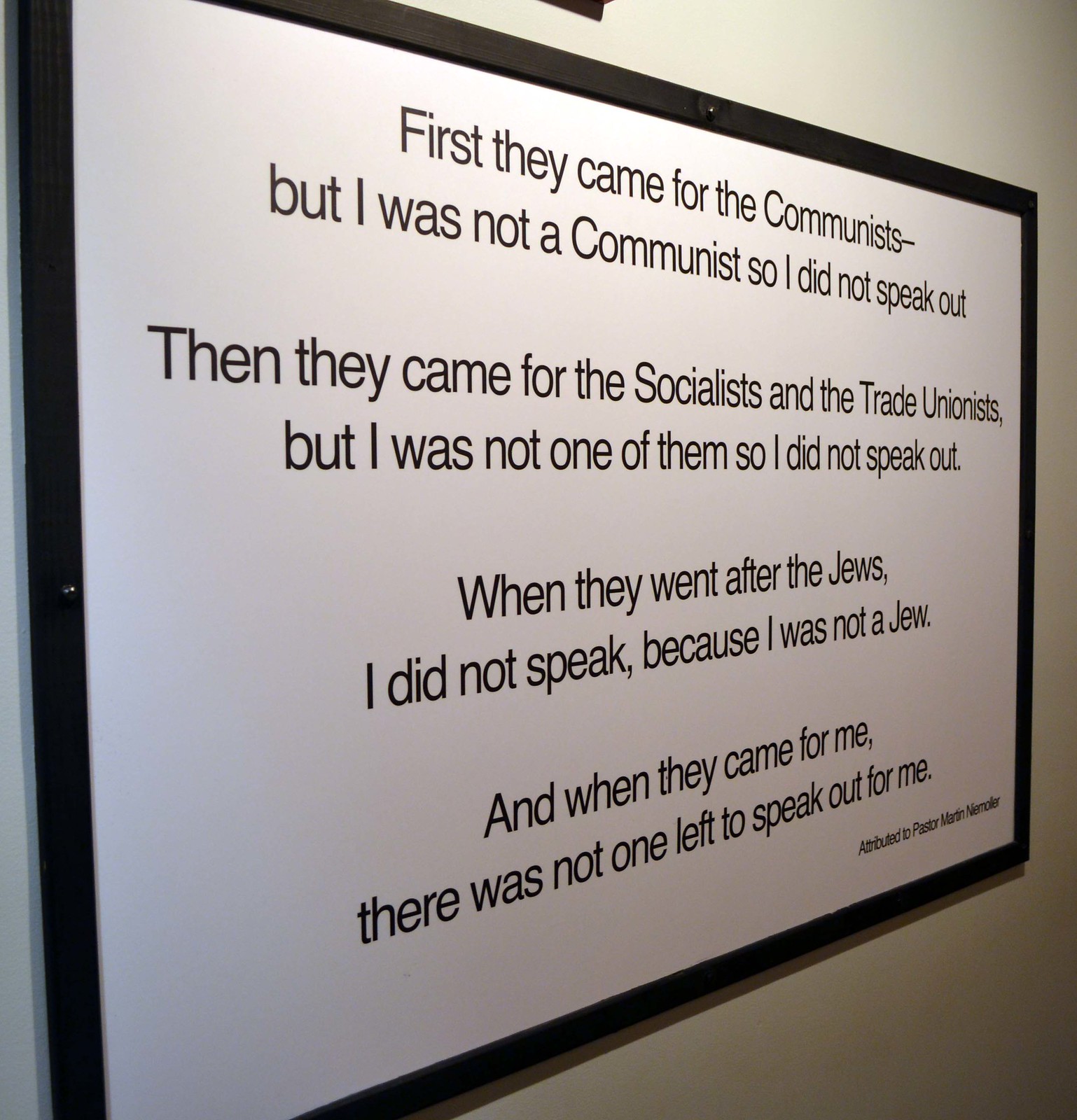The image is a color photograph in a square format, depicting a black-framed, wall-mounted plaque against a white wall. The plaque features a stark, white background with black text that reads, "First they came for the communists, but I was not a communist so I did not speak out. Then they came for the socialists and the trade unionists, but I was not one of them so I did not speak out. When they went after the Jews, I did not speak because I was not a Jew. And when they came for me, there was no one left to speak out for me." The text is attributed to Pastor Martin Niemöller, whose name appears in the lower right-hand corner. Shadows of the plaque cast on the wall suggest it is slightly raised. The upper part of the wall shows a corner, hinting at the possible presence of another unseen poster above the plaque. The perspective of the image is slightly off-center, creating a sense of depth as if looking down a hallway.